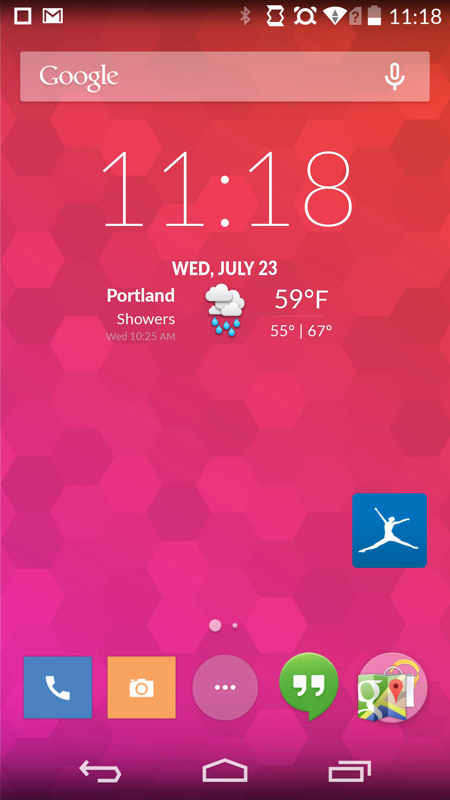A screenshot of a smartphone home screen is depicted. In the upper left corner, there is a white square. Adjacent to it on the right is the Gmail icon. The upper right section displays a series of status icons: the Bluetooth icon, the alarm icon, the Wi-Fi icon, and the battery icon. The current time, 11:18, is also shown in the upper right. Just beneath this, there is a Google search widget featuring the word "Google" on the left in a white area, and a microphone icon on the right within the widget. Directly below the search widget, the time is repeated in a larger, thinner white font, showing 11:18 again. Underneath this, a weather widget indicates the date as Wednesday, July 23rd, and further provides weather details: "Portland, showers, Wednesday 10:25 AM."